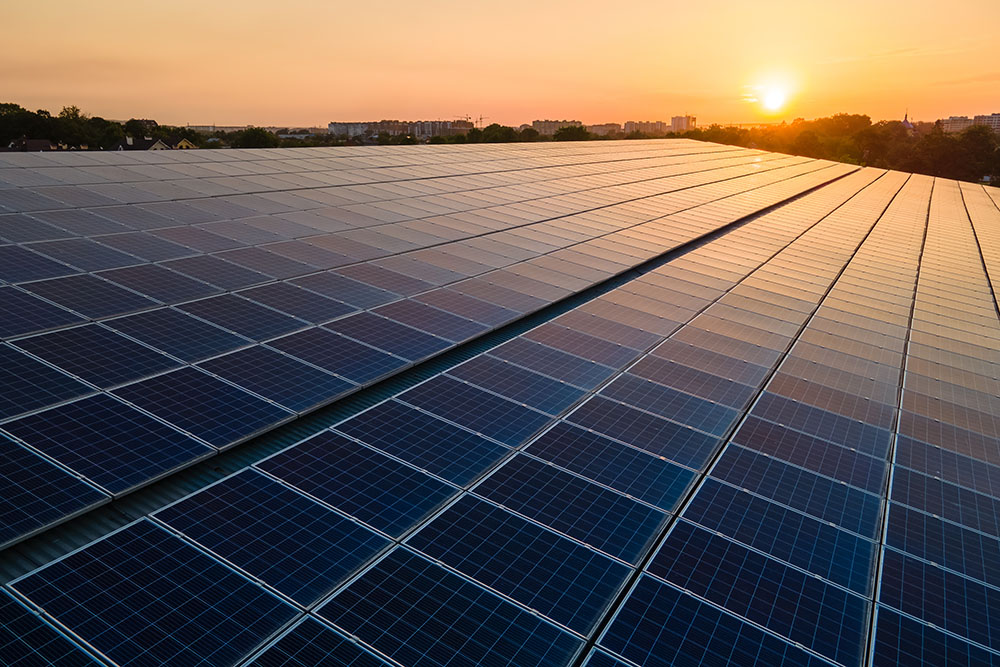The full-color photograph, taken outdoors either at sunrise or sunset, captures a detailed and vibrant scene. The top 20% of the nearly square image showcases an orange-tinted sky with scattered clouds, through which the sun shines. Below this expansive sky lies a community, with indistinct buildings stretching across the frame. The focal point is a vast array of solar panels, bathed in sunlight. It's not clear whether these panels are on rooftops or independent, but there are dozens upon dozens of them. The backdrop includes a hint of a bustling city and trees, underlining an electric and sustainable focus in the scene.